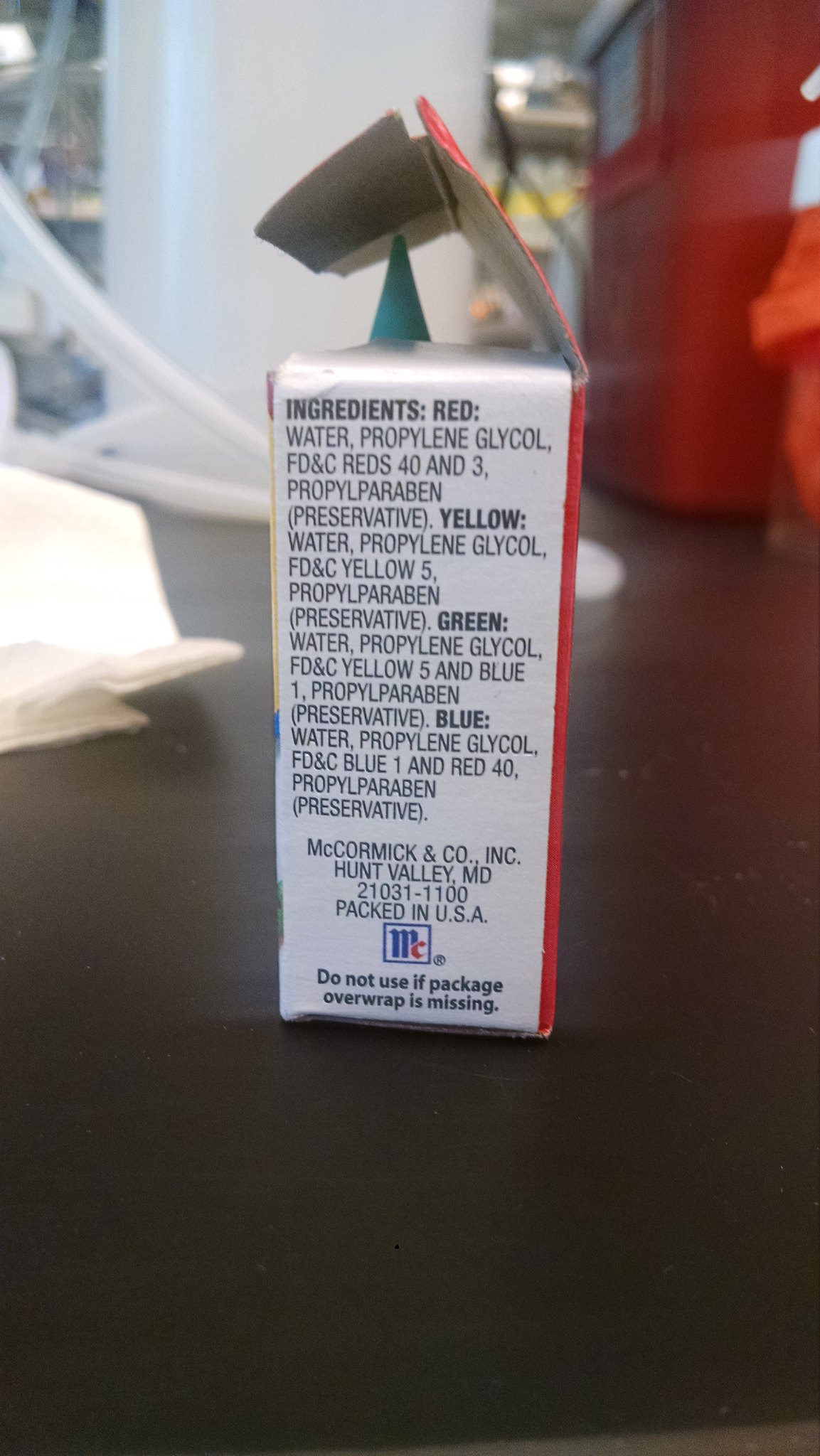In this photograph, an open red box of McCormick & Co. Inc. spices is prominently featured, viewed from a side angle that allows the ingredients list to be seen. The red box has its lid open, forming a distinctive upside-down triangle with one side cut off due to the flap hanging over. The box displays the McCormick & Co. Inc. name, located in Hunt Valley, MD, USA, alongside a blue and red "MC" logo. A cautionary note states, "do not use if packaging overwrap is missing." Emerging from the open lid, a bluish-green cylinder is visible, though it's unclear whether it is inside the box or positioned behind it. The setup rests on a dark brown counter. In the background, there is a red bin to the right and a white pillar at the center. The distant background is slightly blurred, giving the impression that the scene is set in a kitchen. The surface of the counter shows signs of wear with noticeable scuff marks.